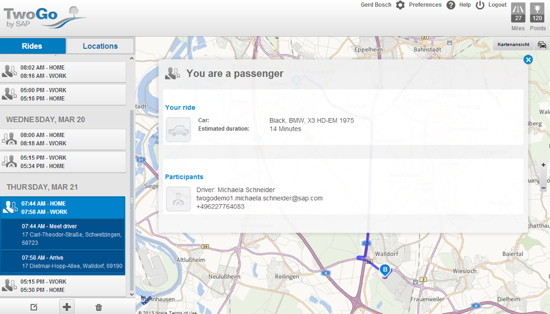This rectangular image, likely taken from a mobile app or a website, features a clean, user-friendly interface. At the top, there's a horizontal gray banner extending across the entire width. On the top left, the word "two" is displayed, with "T-W-O" in gray and "G-O" in blue, just below the phrase "by SAP" in gray. To the right of "two," there is a small graphic showing a road, consisting of one gray line and one blue line, with a tree in the distance.

To the right of this graphic, a series of options is presented: a gear symbol labeled "Preferences," a question mark for "Help," an option to "Log Out," and two small gray boxes with unidentified symbols and numbers. As we move down the image, it is divided into two main sections.

On the left, there is a vertical column titled "Rides and Locations." In this column, "Rides" is highlighted with a blue box and white text, while "Locations" is displayed with a white box and blue text. Below are icons representing people, indicating times for "Home" and "Work."

On the right side of the image, there is a map displayed with a pop-up window overlaying part of it, providing geographical context and potentially specific directions or information. This image depicts details for Wednesday, March 20th, rounding out the comprehensive and informative display.